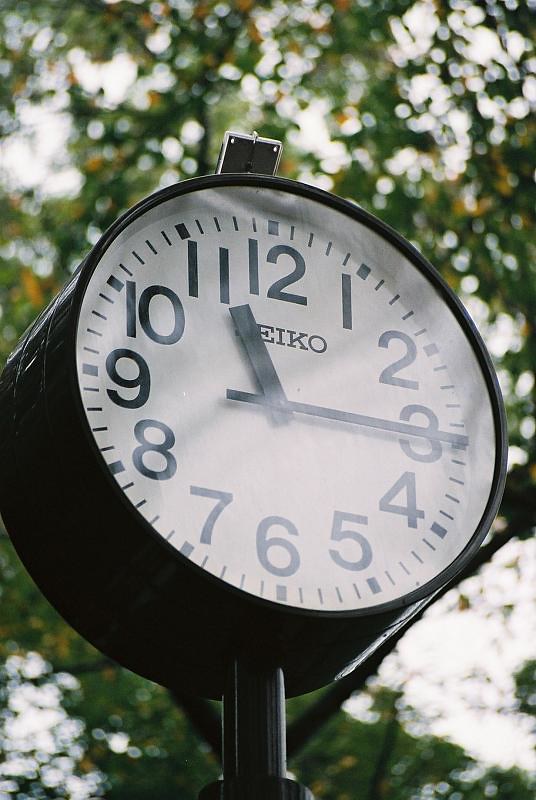In this outdoor scene, we see a large, round Seiko clock prominently displayed atop a sleek black iron pole. The clock face is white, featuring clear, bold black numbers ranging from 1 to 12, with black hands indicating the time as 11:15. Just beneath the 12 o'clock position, the brand name "Seiko" is inscribed. The clock's casing is painted black and appears shiny, reflecting some light. The background is dominated by lush green trees with canopies allowing patches of sunlight to filter through, set against a light blue sky. This well-crafted timepiece serves as a striking focal point amidst the natural setting, combining functionality and elegance.